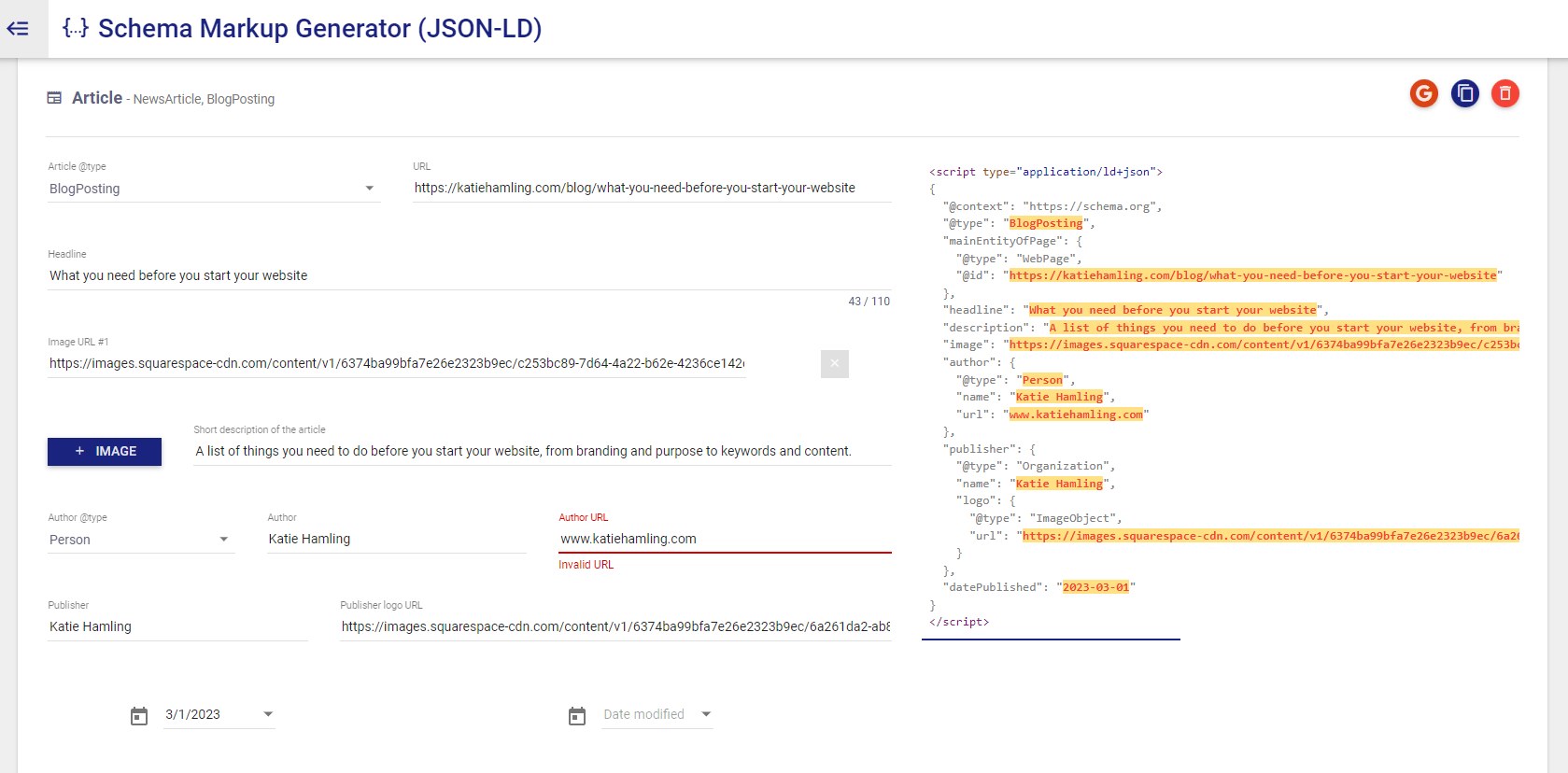This image is a cropped screenshot of a Schema Markup Generator interface in JSON-LD format. At the top left corner, there is a prominent caption in large purple font that reads "Schema Markup Generator," with "JSON-LD" noted parenthetically. Directly beneath this title, the word "Article" appears in smaller gray font. Below this, lines of code and web addresses are displayed.

In the central area of the interface, there is a notable purple button on the left side labeled "Image." At the bottom left, a drop-down box is visible, displaying a calendar date set to "03-01-2023." Adjacent to this is another calendar box that remains unset. On the right side of this section, it shows the "Page Code." The entire interface is set against a white background.

This panel is designed to facilitate the addition of structured data to a website, thereby aiding search engines in better comprehending the webpage content, which in turn can enhance the website's appearance in search results. Essentially, it adds microdata to the HTML of the website to help improve search engine rankings.